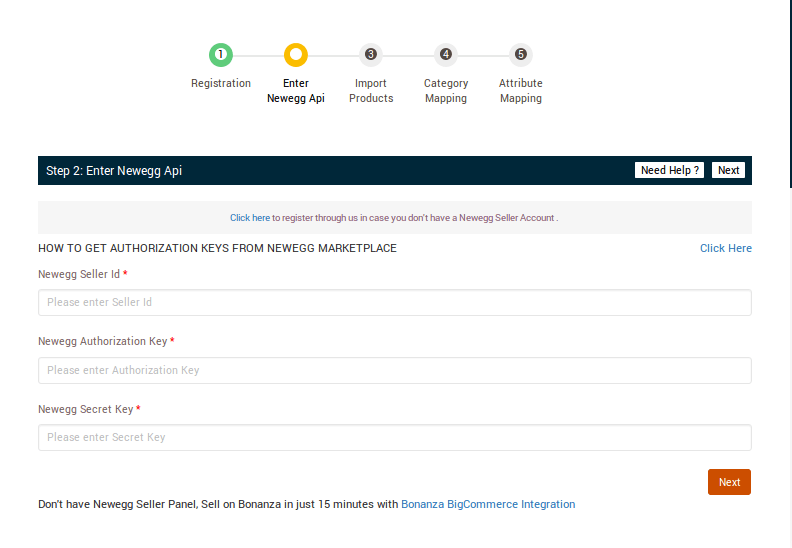### Detailed Caption:

The image depicts a step-by-step instruction interface primarily set against a white background. 

#### Section 1:
- **Left of center**: 
  - A green circle with a black number "1" inside.
  - Directly below the circle, the word "Registration" is written in gray text.

#### Section 2:
- **To the left**: 
  - A yellow circle with a smaller white circle nestled inside.
  - Below this, the black text reads "Enter NEWEGG IAP".

#### Section 3:
- **Progress Steps**:
  - Three consecutive steps labeled "3", "4", and "5", each displayed within a black circle featuring gray numbers.
  - Beneath each circle, actions to be taken are listed in gray text:
    - "Import Products"
    - "Category Mapping"
    - "Attribute Mapping"

#### Section 4:
- **Step Highlight**:
  - A section with a black background and gray text that states, "Step 2: Enter NEWEGG IAP".

#### Section 5:
- **Right side**:
  - Two white boxes with black text in the center. The left box says "Need Help", and the right box says "Next".

#### Section 6:
- **Instructions and Help**:
  - A gray background with darker gray text stating: "Click here to register through us in case you don't have a NEWEGG seller account".
  - Contrasting sections with black background and white text alongside white background and black text:
    - Instructions: "How to get authorized keys from the NEWEGG marketplace" with "click here" in blue text next to it.
    - Fields for user input:
      - "NEWEGG Seller ID" followed by a space to enter the ID.
      - "NEWEGG Authorization Key" followed by a space to enter the key.
      - "NEWEGG Secret Key" followed by a space to enter the secret key.

- **Footer Message**:
  - In black text: "Don't have a NEWEGG seller panel?"
  - Followed by: "Sell on Bonanza in just 15 minutes with Bonanza Big Commerce integration," where "Bonanza Big Commerce" is highlighted in blue text.

#### Final Section:
- **Call to Action Button**:
  - An orange button located on the right-hand side with the word "Next" written in white.

This detailed breakdown provides a comprehensive view of the interface as shown in the image.